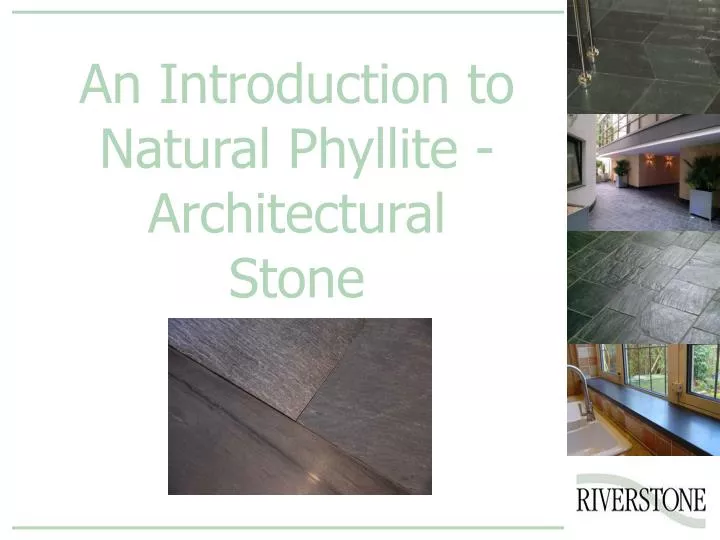The image appears to be a detailed PowerPoint slide or an advertisement for natural phyllite architectural stone. The main section, covering the left two-thirds of the slide, features text in light green that reads "An Introduction to Natural Phyllite - Architectural Stone." This text is framed by light green horizontal bars at the top and bottom. Directly beneath this title, there is a close-up photograph showcasing three pieces of phyllite stone tiles in varying shades and textures: dark brown, gray, and beige, closely placed together.

On the right side of the slide, four vertically arranged images illustrate different use cases of the stone tiles. The top image features a close-up of smooth, dark gray stone tiles with metal poles. The second image shows a building exterior with a stone-tiled corridor, flanked by large plants and gray stone steps leading up to it. The third image provides a detailed view of rough-textured gray stone tiles. The fourth and final image depicts a kitchen scene with dark gray stone countertops atop wooden cabinets, a silver faucet, and a white washbasin.

In the bottom right corner of the slide is a logo comprised of a light green swirl with the text "RIVERSTONE" in black capital letters below it. This detailed layout offers a comprehensive visual and textual introduction to the natural phyllite architectural stone, highlighting its versatility and aesthetic appeal in different settings.